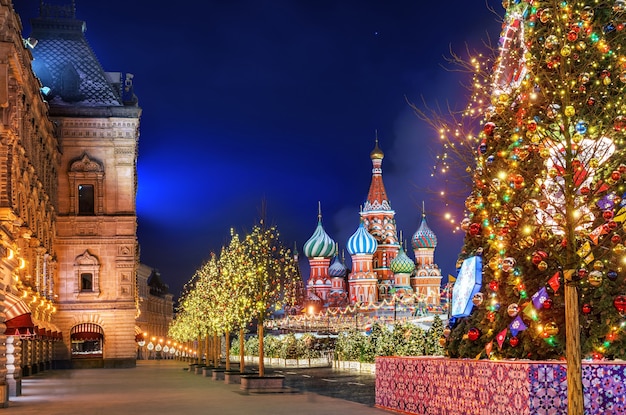The photograph captures a festive Christmas display set against the backdrop of an ornate, historical setting, likely in a foreign country such as Russia. Dominating the foreground to the right is a beautifully lit and brightly decorated Christmas tree, adorned with colorful ornaments and sparkling lights that stand out vividly against the night sky. Not far off, smaller, non-Christmas trees add depth to the scene.

The focal point of the image is a collection of iconic, teardrop-shaped buildings, painted in an array of vibrant colors like blue, green, and red, reminiscent of classic Russian architecture, specifically invoking the imagery of Saint Basil's Cathedral with their whimsical, candy-like domes. These structures, grouped together, create a striking, almost cartoonish contrast to the surrounding architecture. To the left of the image, there's an ornate building with a dark blue roof, its tan facade adding an elegant touch to the holiday spirit permeating the scene.

Overall, the display, likely set up specifically for the holidays, blends the timeless charm of historical architecture with the festive exuberance of Christmas decorations, creating a mesmerizing and vibrant nighttime tableau.